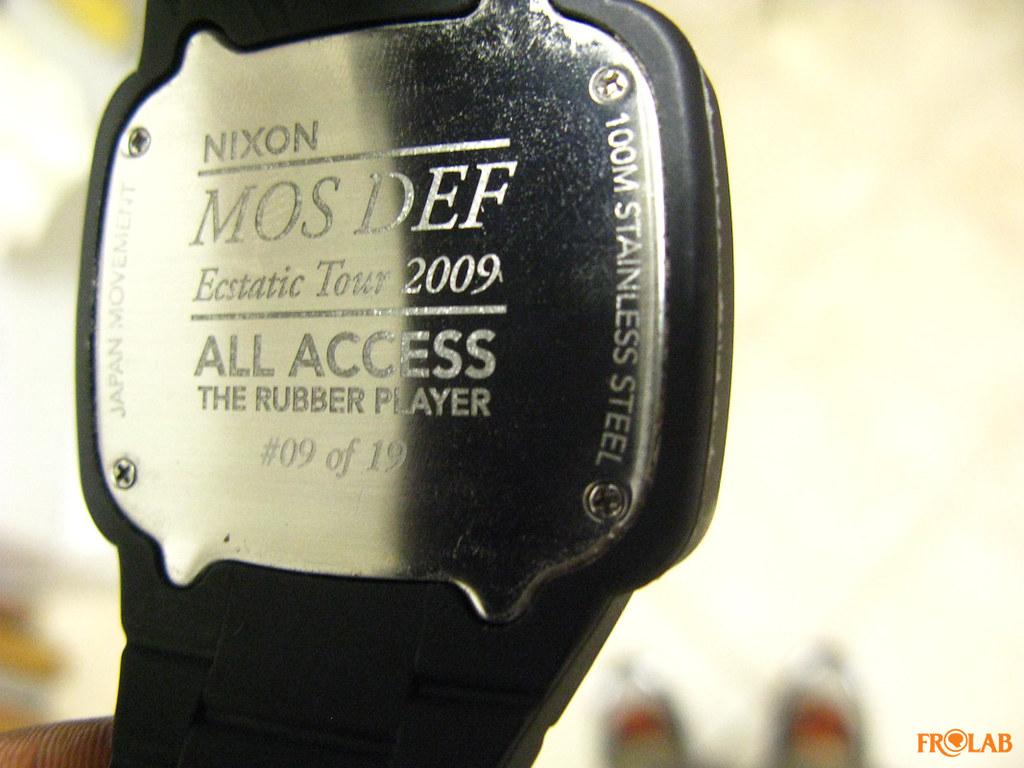The image depicts the back of a black wristwatch with black straps. The stainless steel backplate of the watch, which appears to resemble a silver badge, features several engravings. Prominently, it reads "Nixon" horizontally along with "Mos Def," "Ecstatic Tour 2009," "All Access," "The Rubber Player," and "#09 of 19." Additional text includes "Japan Movement" and "100M Stainless Steel" vertically on the right-hand side. At the bottom right, there's a logo that reads "FroLab." The background of the picture is an ivory color, and the image is presented in a horizontal, rectangular format.